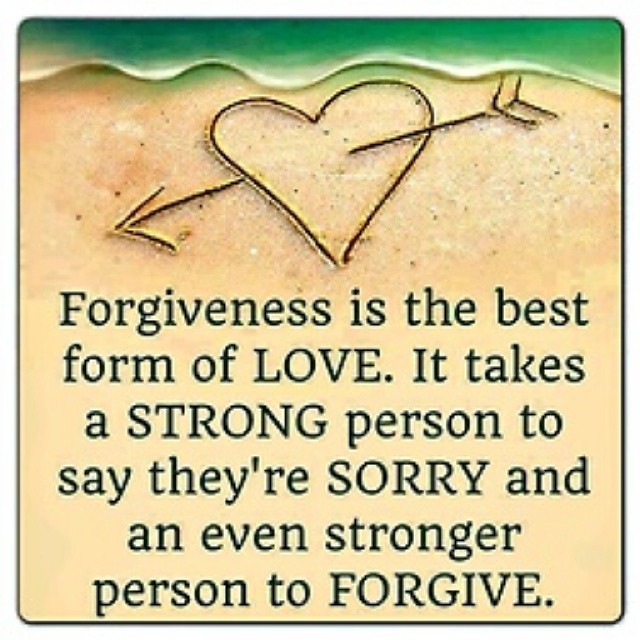The image features an inspirational quote superimposed on a color illustration of a sandy beach scene. The sandy beach occupies the bottom seven-eighths of the image, with a hand-drawn heart pierced by an arrow centered towards the top of the sand. Above this, the top eighth of the image displays dark green and bluish-green ocean water with white foam at the shoreline. The heart, drawn as if with a finger, points to the left with feathers on the top right of the arrow. The text is in a dark color and reads: "Forgiveness is the best form of love. It takes a strong person to say they're sorry and an even stronger person to forgive." The quote is centrally aligned beneath the drawing, making up a significant portion of the composition. This square-format illustration combines elements of graphic design and typography, making it suitable for social media sharing, particularly on platforms like Facebook.